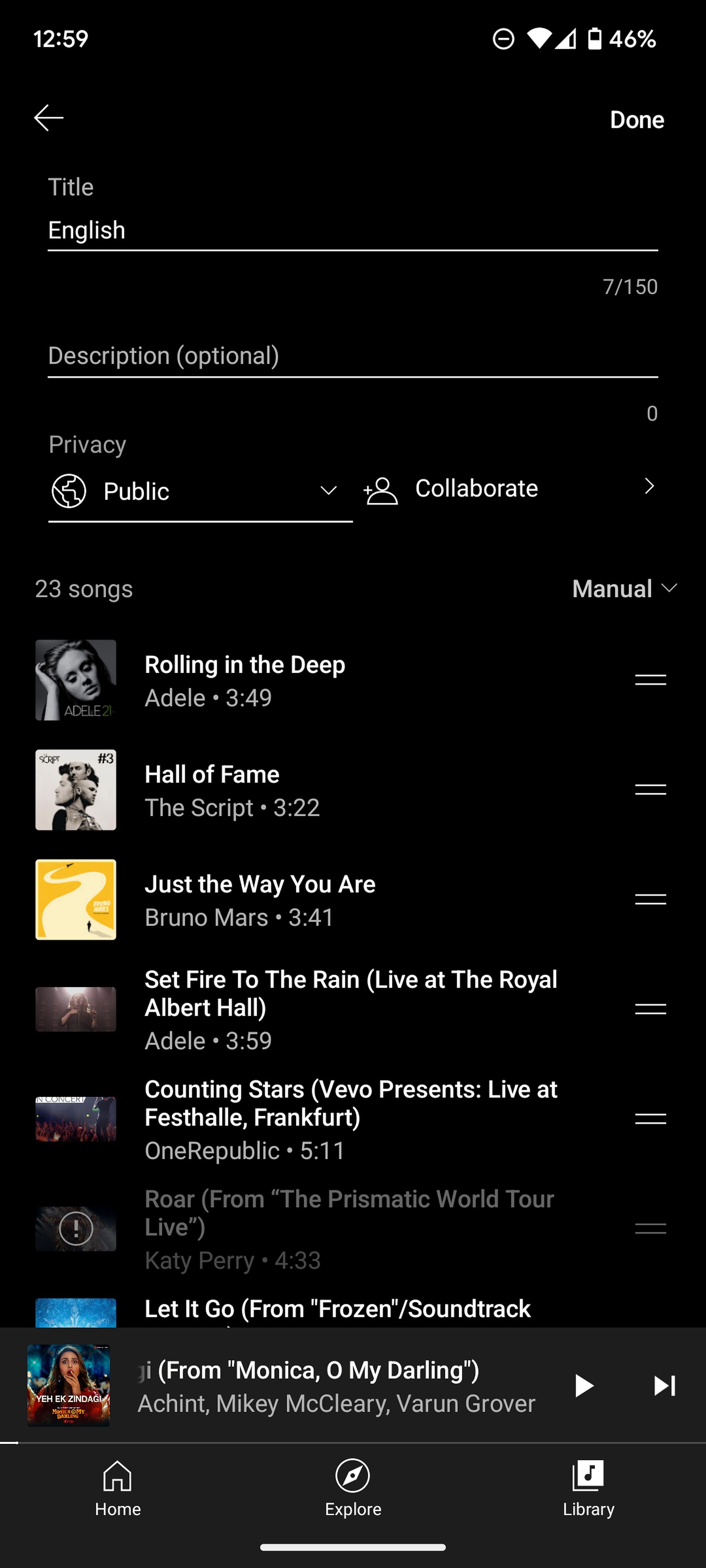Here is a cleaned-up and detailed caption for the described screenshot:

---

The mobile screenshot appears to be from a music app, displayed on a device with a current time of 12:59 indicated in white text at the upper right corner. The top-left corner of the screen features a white circular icon with a central dash, likely representing some control or status indicator. Adjacent to this icon are the Wi-Fi signal symbol showing nearly full bars, and a battery icon displaying approximately 50% charge. To the right of these icons, "46%" is shown in white font.

Towards the top-left of the image, there's a light gray arrow pointing left, serving as a back navigation button. On the opposite end at the top-right, “Done” is written in white text, likely a button to finish or save actions.

Under the header section, the word "Title" is written in gray, followed by an editable text area displaying "English" in white text. This area appears to be underlined in white, and towards the bottom right, it shows "7/150" in light gray, indicating characters used out of a max limit.

Beneath this, the label "Description (optional)" is present in gray text. There is another underlined area here, with a light gray "0" at the bottom right, suggesting space for additional text input.

Further down, the label "Privacy" is displayed in light gray, with a large white globe icon and the word "Public" in white, indicating the current privacy setting. This setting includes a downward-facing arrow to the right, suggesting it is a dropdown menu.

Towards the right, there is a user icon with a plus sign near the neck, labeled "Collaborate" in white text, with an arrow pointing right, indicating a submenu for collaboration options. Finally, it states "23 songs" in gray on the left, and "Manual" in bold white text to the right, accompanied by a downward-facing arrow, indicating playlist settings or sorting options.

---

This detailed caption captures all elements described and conveys a clear visual of the interface.